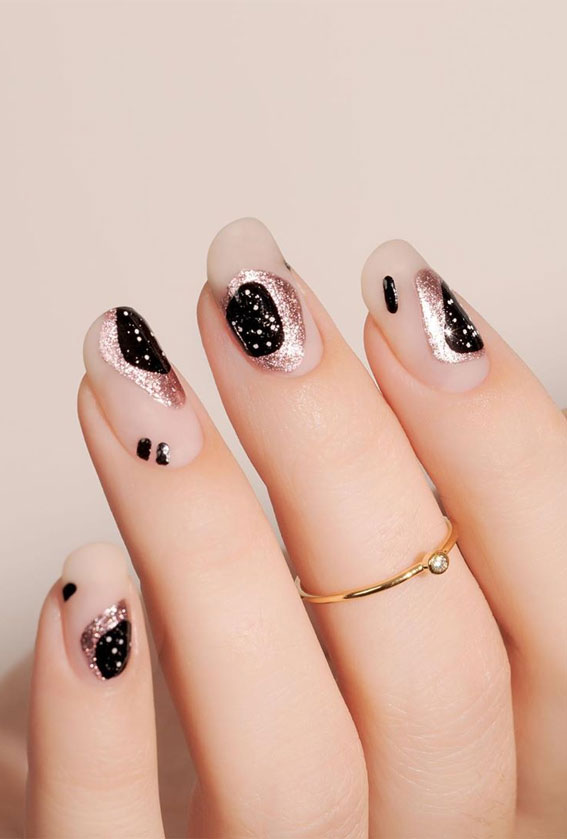This photograph showcases the four fingers of a woman’s left hand, positioned vertically against a faint pinkish-gray background with an emphasis on the nails' intricate designs. The woman, who appears to have light-colored skin, possibly Asian or white, wears a delicate thin gold ring with a clear diamond on her middle finger, situated just above the main knuckle. Each fingernail is adorned with a base of cloudy white or pink polish. On the nails, there are decorative elements: a prominent shiny pink blob overlaid with a sparkly black blob, complemented by scattered black marks and gold speckles, creating an abstract, whimsical look. The background of the image, resembling a beige or light pink wall, subtly enhances the visual appeal of the painted fingernails. Only the fingers up to where they begin are visible, with no sight of the thumb, making the nail art the central focus.